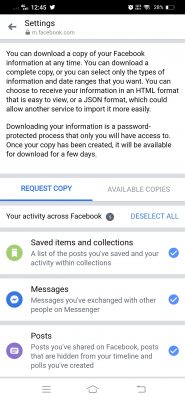The image, captured from a smartphone, displays a section of the Facebook settings menu. The screen shows the option to download a copy of one's Facebook information. The specific URL displayed is mfacebook.com. The settings section explains that users can download a complete copy of their Facebook data or select specific types of information and date ranges. Users can choose between receiving their information in HTML format for easy viewing or JSON format, which facilitates importation by other services. The process of downloading this information is password-protected and accessible only to the user. Once the data copy has been created, it will be available for download for several days. A blue-highlighted and underlined 'request copy' button is prominently featured, indicating that the user has clicked on it. To the side, there is also an 'available copies' section. Further down the screen, there are categories such as saved items in collections, messages, and posts, each marked with a blue circled arrow. These arrows indicate expanded menus for these categories.